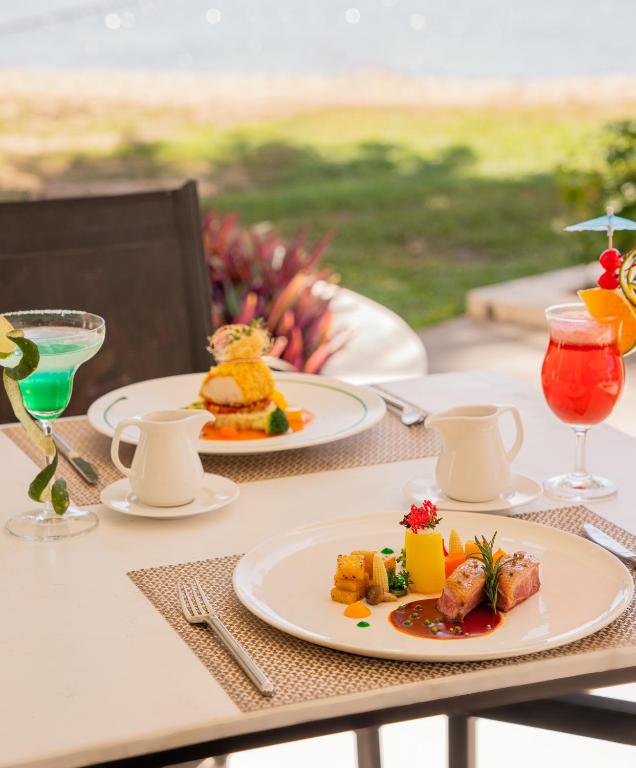This image features a detailed outdoor patio scene set for a meal, possibly lunch or dinner. In the background, a lush, green lawn stretches towards a body of water, which remains out of focus. In the foreground, an outdoor dining table—cropped at the edges—hosts a meticulous setup. The table itself is brown with a beige top and is surrounded by brown chairs, with one chair partially visible near the lower right corner of the image.

The table is adorned with beige and brown place settings, including white plates, and appears to be set for two. Notable items include a saucer and a creamer at each setting. Two plates of food are prominently displayed: the nearer plate appears to feature a seared tuna with pineapple, and the farther plate seems to contain a hamburger slider. Each plate is accompanied by vegetables and sauces, adding to the visual appeal.

Additionally, the table is graced with two distinctive cocktails: on the right, a red drink garnished with an umbrella, an orange slice, and two cherries; on the left, a green drink decorated with a lime wedge, partially wound around the glass stem. Standard cutlery, including a fork and knife, completes the table setting, preparing it perfectly for an inviting meal.